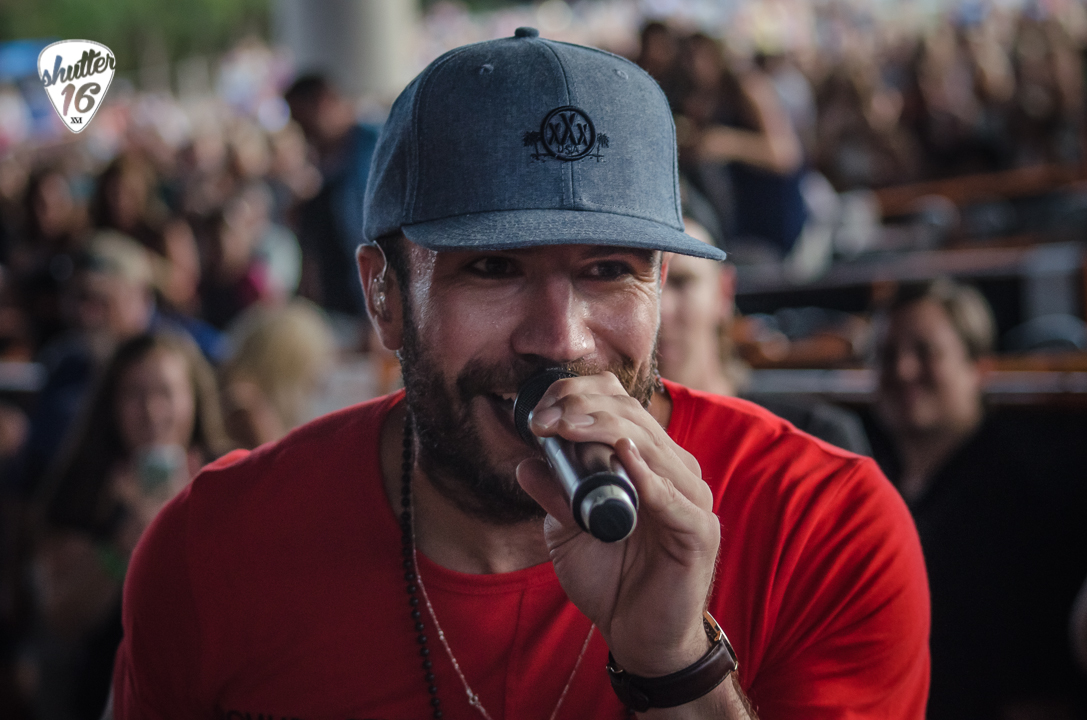This horizontally-aligned rectangular photograph features a man speaking into a silver microphone with a black bottom, held in his left hand, while facing slightly to the right. The man is wearing a denim-looking gray baseball cap with a circular logo on the front that reads "XXX" in black, with "USA" under it. He has a short brown beard, a red t-shirt, a brown watch on his wrist, a long set of black beads, and a thin silver chain around his neck. His expression is deeply engaged, suggesting he might be singing or rapping with considerable emotional effort. Behind him, a blurred audience is visible, likely seated on bleachers that slope upwards on the right side of the image. In the upper left corner, there is a guitar pick-shaped logo with cutout letters that read "Shutter 16" against a white background.